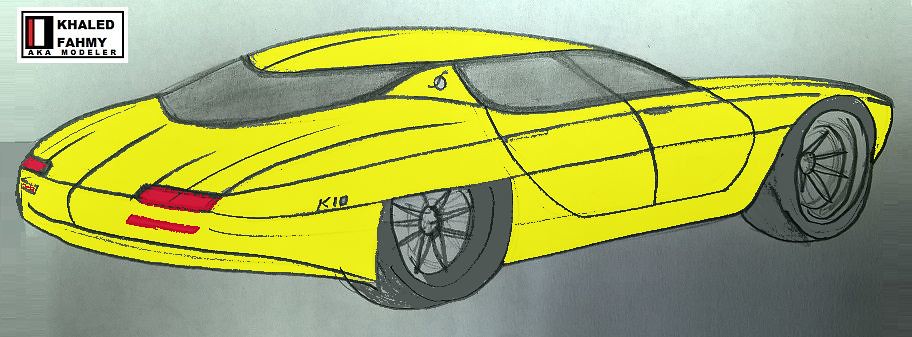The image is a detailed color drawing of a lemon-yellow sports car, reminiscent of a Corvette, flaunting a sleek, low-to-the-ground body with a rounded top. The drawing appears to be rendered with colored pencils or felt-tip markers on a light grayish-green paper, which fades to a darker shade towards the right-hand corner. The car is depicted in profile, facing the upper right, and features large, spoked wheels with dark gray, chunky tires. 

Notably, the car has tinted gray windows and is labeled “K10” beside the back right wheel. The rear sports prominent red rectangular brake lights. There is also a small emblem resembling a circle with a squiggly line behind the back seat window on the passenger side.

In the top left corner of the image, there is a small flag-like logo comprising horizontal stripes in red, white, and blue, contained within a rectangle. Beside it, the text reads "Khalid Family aka Modeler," suggesting that this is a concept design for a model car.